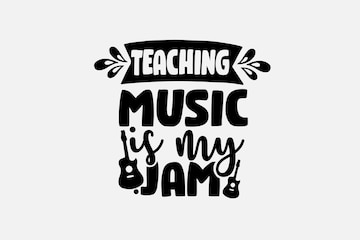In this black-and-white graphic image with a rectangular white background, the central focus is a prominent black banner with a slightly tapered design at both ends. The banner, styled with bubble letters, reads "TEACHING" in white. Flanking the banner are three stylized water drip graphics on each side, also in black and white. 

Below the banner, in thick black print, the word "MUSIC" stands out. Underneath this, the phrase "is my" appears in an elegant, curvy script. Following this, back in the thick black print similar to "MUSIC," the word "JAM" is displayed. The phrase "is my jam" spans across two levels. 

Complementing this text are two black guitar silhouettes, one placed before the phrase "is my" and the other after "JAM." The entire composition underscores a fun and creative visual style using only black and white elements, emphasizing the words with distinct text and playful graphical elements.